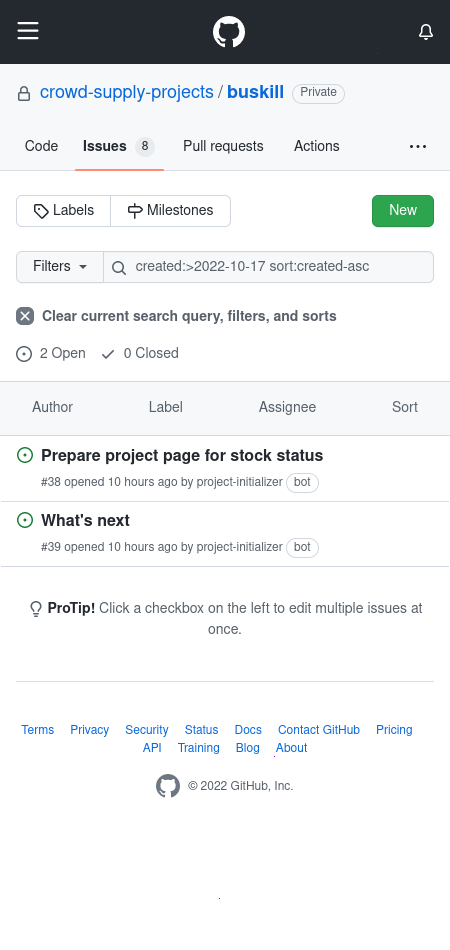This image is a detailed screenshot of a GitHub repository interface as viewed on a mobile phone. At the top, there is a black navigation bar featuring three horizontal lines, a white circle containing a silhouette of a cat, and a bell icon. Below the navigation bar is the repository name "CrowdSupply-Products/Buzzkill" marked as private. 

The main interface displays several tabs: Code, Issues, Pull Requests, Actions, and a menu signified by three dots, with "Issues" being highlighted and underlined in red, and showing a total of eight issues.

Beneath the tabs, there are options labeled Labels, Milestones, and a green button labeled "New". Further down is a section for Filters and Search, accompanied by a box with the text: "Clear current search query, filters, and source", which is checked. Another selection area labeled "To Open" features a radio button, while "Zero Closed" has a check mark.

The interface shows filters for Author, Label, Assignee, and Sort in a gray box. A list follows with tasks marked by green circles, including:

1. "Prepare Project Page for Stack Status," issue #38, opened 10 hours ago by Project Initializer.
2. "What's Next," issue #39, opened 10 hours ago by Project Initializer.

A Pro Tip advises: "Click a checkbox on the left to edit multiple issues at once."

At the bottom, standard GitHub navigation links are displayed in blue: Terms, Privacy, Security, Status, Docs, Contact, GitHub, Pricing, API, Training, Blog, and About.